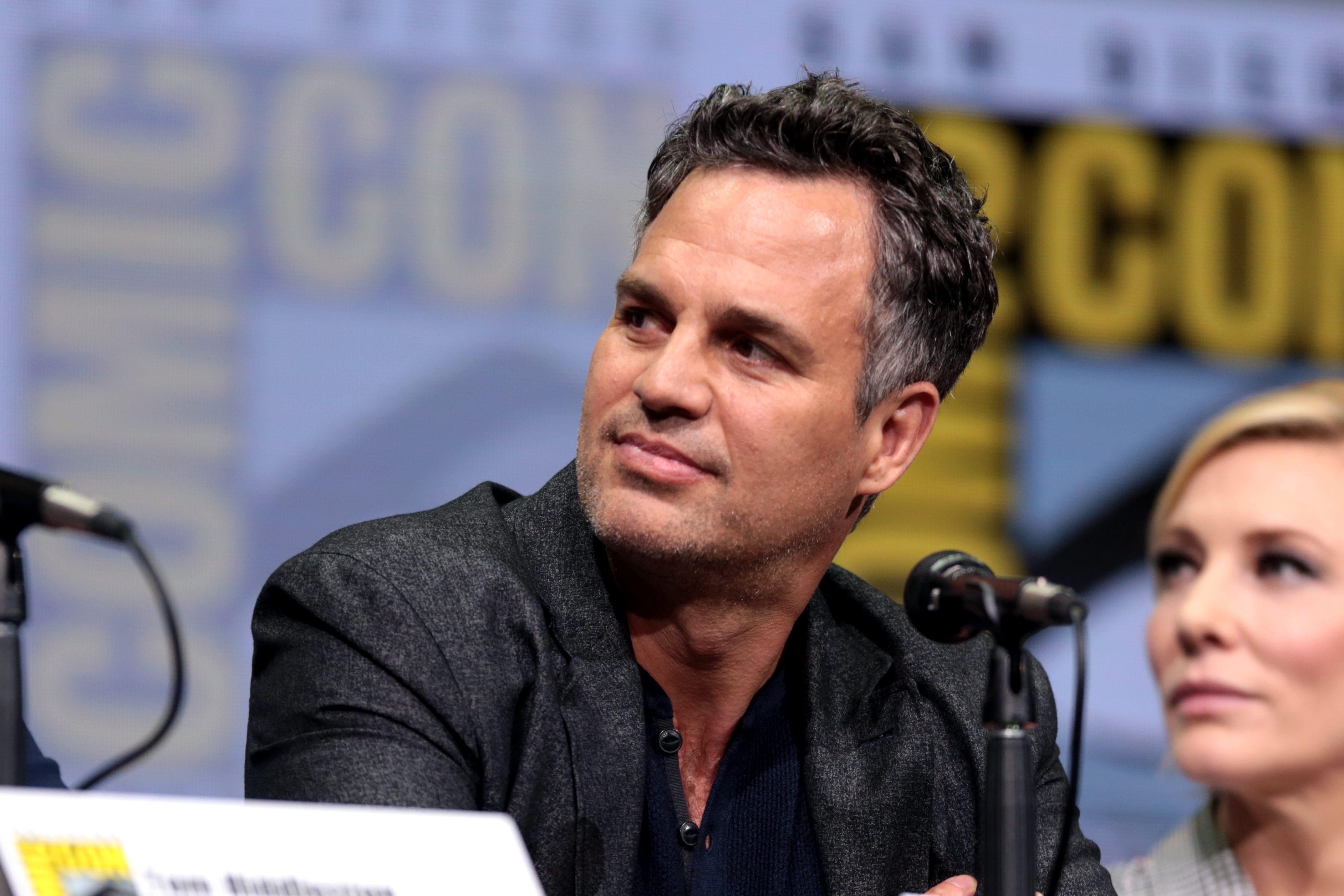The image captures a moment at the San Diego Comic-Con, evident from the white backdrop adorned with "San Diego" in black font at the top and "Comic-Con" in bold yellow, all set against a purple-blue banner. At the center of the photograph is a man with short black hair accented with a hint of white—identified as Mark Ruffalo. He is seated behind a table or a dais, turning his head to his left, where his gaze, along with a slightly out-of-focus woman with short blonde hair in a gray shirt, is directed towards the unidentified person off-camera. In front of Mark Ruffalo is a microphone, partially cropped out on the left side of the image, alongside a name placard, though the name is slightly cropped and out of focus. Mark Ruffalo sports a black shirt and blazer, adding a touch of formality to the scene.